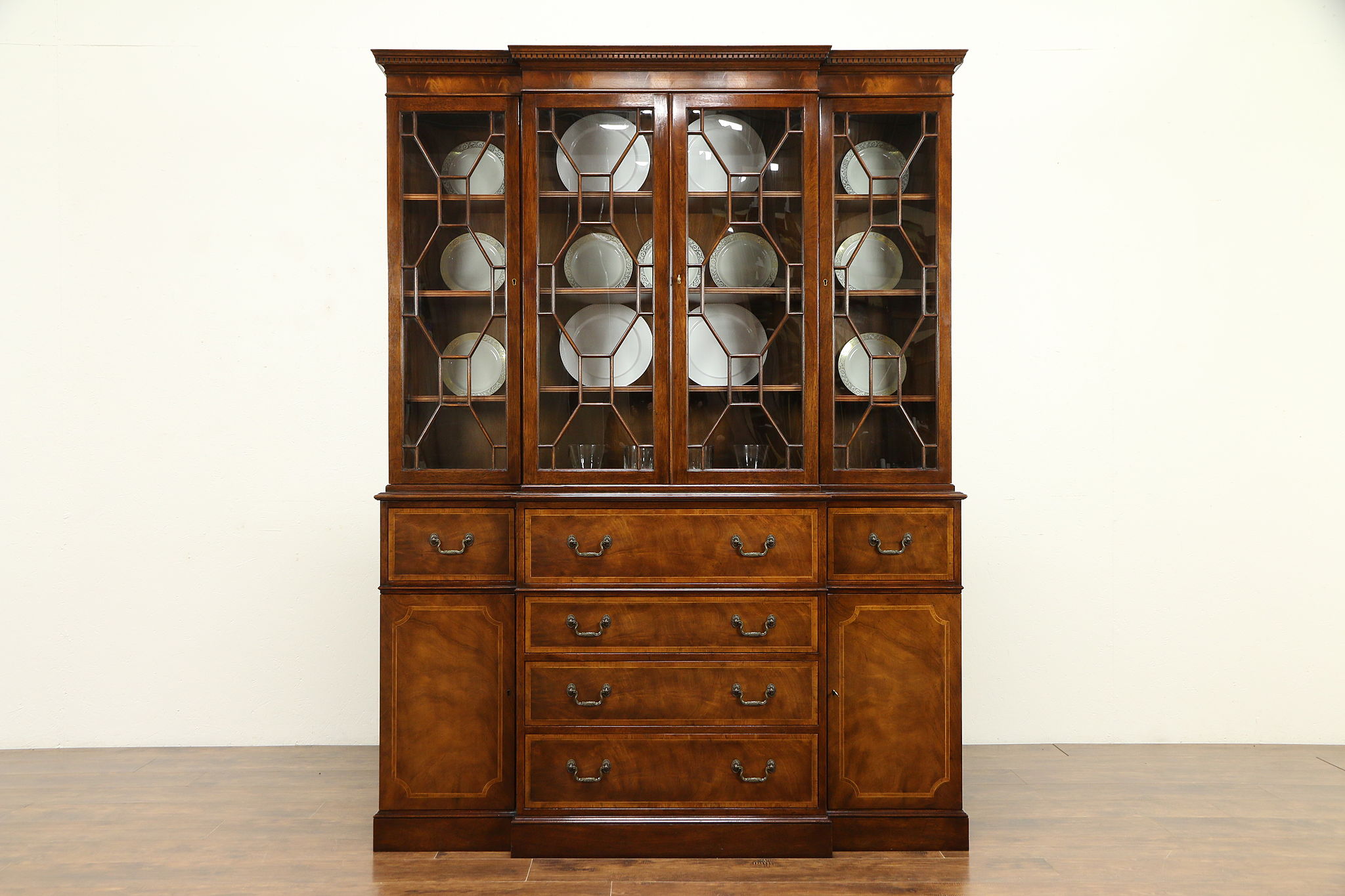This image showcases a large, antique china cabinet made from dark wood, positioned against a white background wall on a smooth, shiny wooden floor with darker brown lines and grooves. The cabinet features multiple sections and intricate details. The top half consists of two glass-fronted cabinet doors, adorned with a pattern of metal inlays and dark-colored, possibly bronze handles, similar to those on the rest of the piece. Inside, it displays four shelves, each garnished with neatly arranged plates—one plate per position, including some that appear to be light blue amidst the predominantly white set.

Below these glass doors, there are four large drawers centrally aligned, each equipped with two matching dark handles. Flanking these central drawers on each side are smaller drawers at the top, also with dark handles, accompanied by long rectangular cabinet doors underneath. The cabinet’s sturdy and ornate design, supported by its polished wooden floor setting, adds to its vintage charm and elegance.